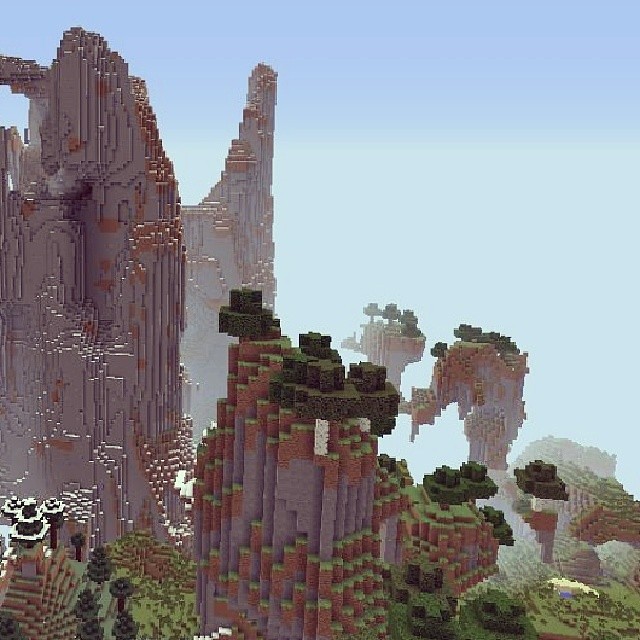A detailed screenshot from the popular game Minecraft showcases various block structures in a scenic landscape. On the left side, a towering mountain made of brown blocks with darker bricks embedded within stands prominently, showcasing the game's signature blocky aesthetic. Another similar-sized mountain appears in the background, slightly obscured by a misty atmosphere that gives depth to the image. In the foreground, a structure adorned with green, plant-like blocks can be observed, adding a touch of life to the otherwise rugged terrain. The sky transitions from a deeper blue at the top to a lighter, mistier blue towards the horizon, enhancing the mystical ambiance of the scene.